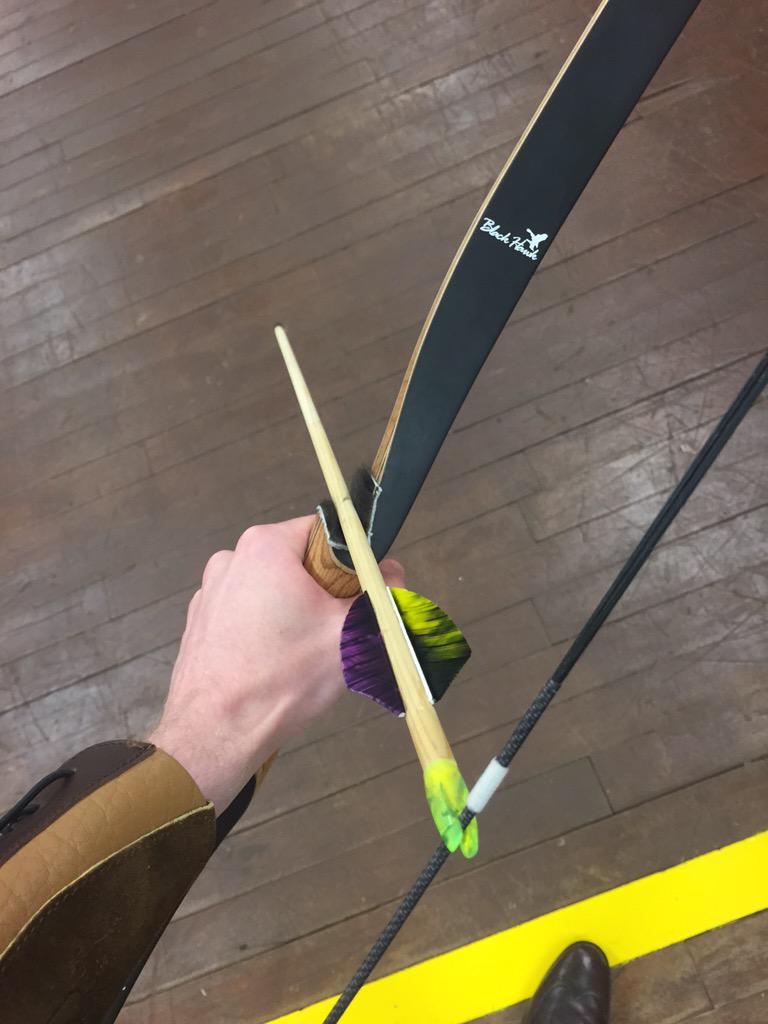The image features a person holding a sleek, black bow with brown handles. The bow is adorned with some white lettering, partially visible, and appears to read "Black" followed by an indistinguishable word. The person is also holding a brown arrow with striking purple fletching and additional feathers in shades of lime green, yellow, and gray. The fletching at the back of the arrow features green-edged tips, designed to fit snugly against the string of the bow.

The archer is wearing a dark brown and light brown sleeved jacket, and has a fair complexion. Their hand firmly grips the bow, ready to take aim. The background reveals a gray, wood-paneled floor with a distinct yellow line running across the bottom of the image. A foot, clad in what seems to be a brown or black shoe, stands aligned with this yellow line, indicating the archer's stance.

The bow itself has a brown edging where the arrow rests, featuring a small L-shaped notch to secure the arrow in place. The overall focus of the image is on the poised bow and arrow, suggesting the person is about to release the arrow towards a target.